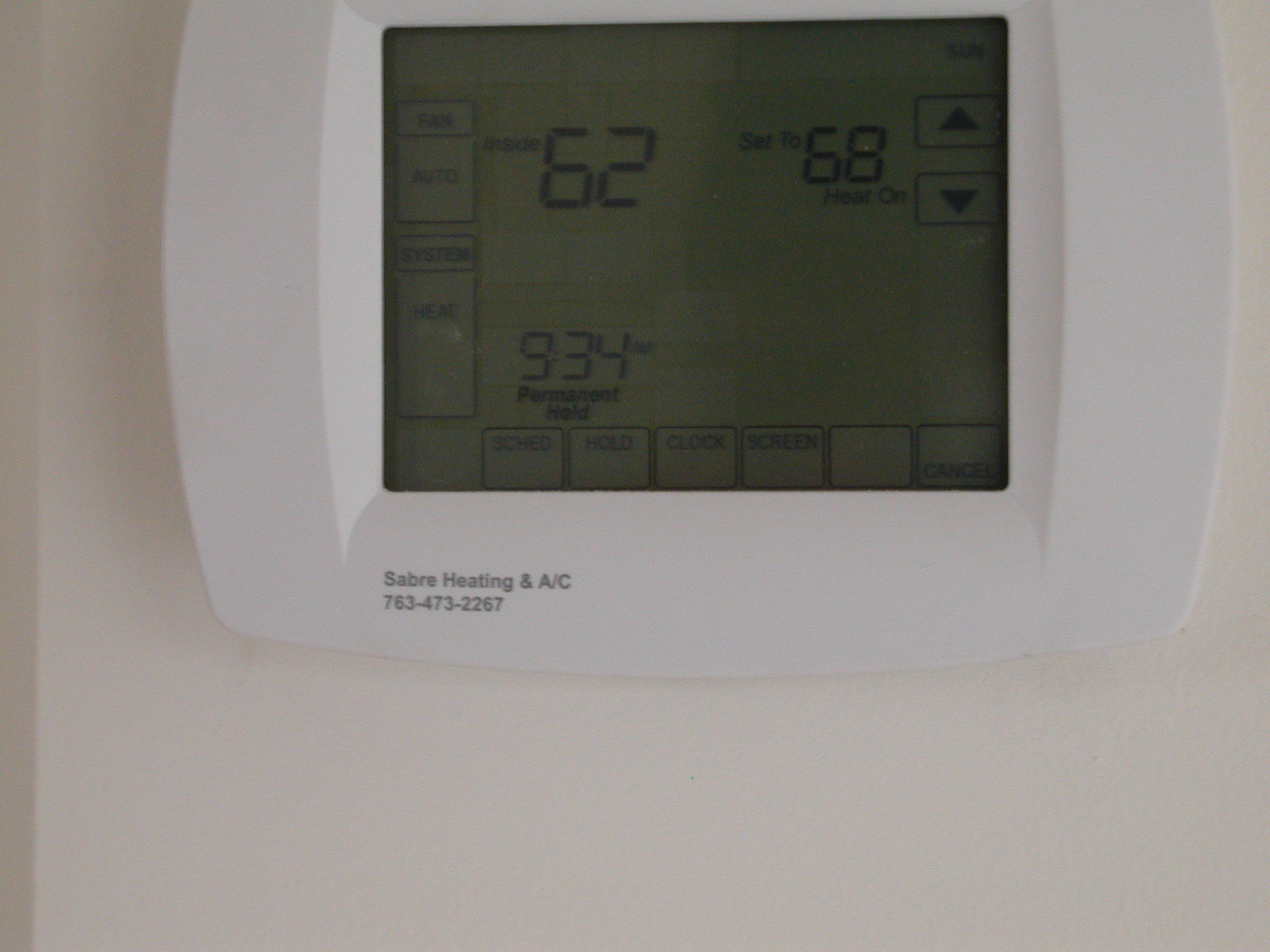The image depicts a meticulously painted white wall. Mounted on the wall is a white thermostat, prominently displayed. The thermostat measures approximately 6 to 9 inches in width and 5 to 7 inches in height. Surrounding the display is a white rectangular frame. The thermostat is branded with "Sabre Heating and AC" along with the contact number "763-473-2267".

The digital display on the thermostat is active but not brightly illuminated. The top line of the display reads "Fan/Auto", "62", "Set to 68", and "Hold On" from left to right. Below this, there are up and down arrows for adjusting the temperature. The subsequent line shows "System Heat" followed by the time "9:34", without indicating whether it is AM or PM. Just beneath, it says "Permanent Hold".

At the very bottom of the display, a row of buttons with various functions is visible. These buttons are labeled "Sched" for schedule, "Hold", "Clock", "Screen", an unlabeled blank button, and "Cancel". Overall, the image offers a close-up view of the thermostat designed to regulate heating and cooling systems.